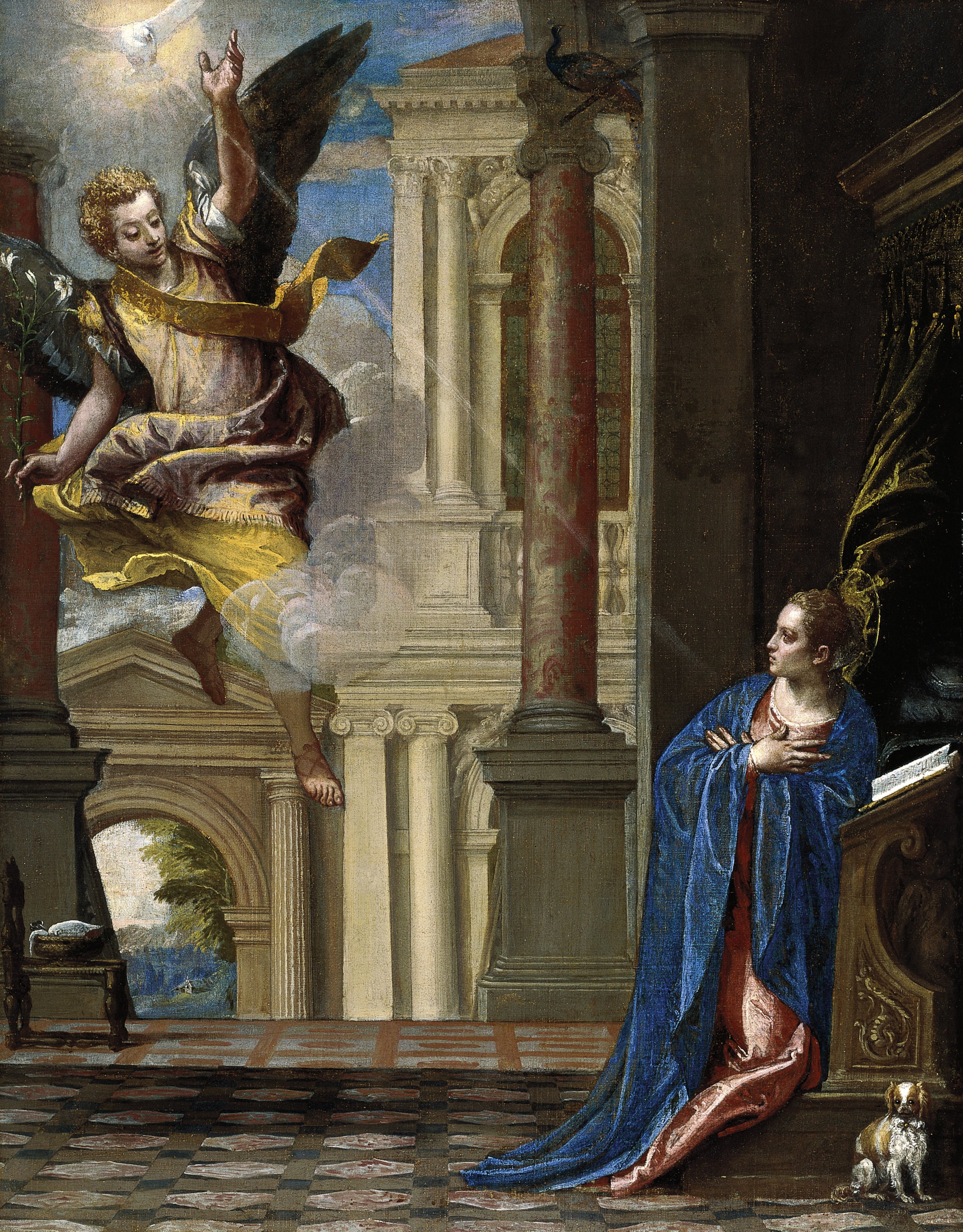The painting depicts a classical scene set against the backdrop of Roman architecture, featuring grand columns, a tiled forum-like floor, and an opulent multi-storied building. At the center, a young, fair-skinned woman with brown hair is dressed in a blue robe over a red gown, leaning on a pulpit or column on the right side of the image. At her feet sits a small toy dog. In the upper left, a male angel with golden hair and black wings appears, dressed in a golden robe. The angel extends one arm upwards towards a glowing white dove that emits radiant light, casting beams down on the scene below. The angel is surrounded by clouds, and his gaze is directed towards the woman. The detailed setting and rich symbolism give the painting a sense of divine intervention and celestial presence.